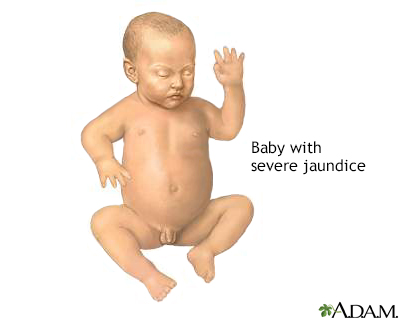The image is a detailed, realistic illustration of a naked, male newborn baby displayed against a white backdrop, likely from a medical journal. The baby has short black hair, long pointed ears, and is depicted with a slightly yellow skin tone, indicative of severe jaundice, as noted by the text to the right that reads "Baby with Severe Jaundice." The baby's left arm is raised with its fingers extended, while its right arm is down by its side, with elbows slightly cocked back and feet in a crouched position. At the bottom right corner of the image, there is a green logo resembling a clover leaf with five petals next to the text "A.D.A.M." in black. The baby’s eyes are closed, and it appears to be looking down to its right-hand side.